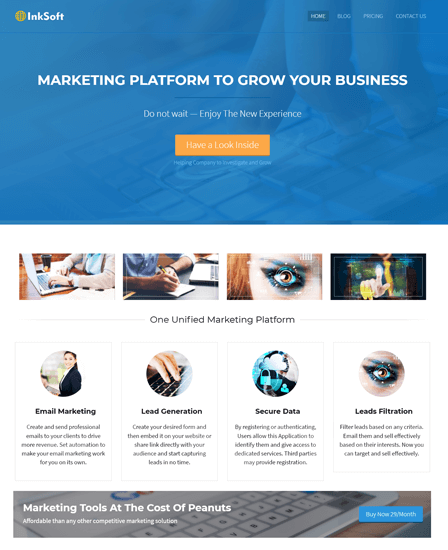A screenshot of a marketing website is displayed. The top section of the page features a blue background. On the top left, the word "InkSoft" is written in white, accompanied by a circular yellow logo to its left. On the right side of this top section, there are four navigation buttons labeled "Home," "Blog," "Pricing," and "Contact Us." Below this navigation bar, white text reads "Marketing platform to grow your business," followed by an invitation to "Do not wait, enjoy the new experience." An orange button with the call to action "Have a look inside" stands prominently with white text.

Beneath the blue header is a white section. At the top of this section, there are four images: one depicting someone typing on a laptop, another showing a person writing a note on paper, a close-up of an eye with a diagram over it, and an image of a hand surrounded by glowing lights.